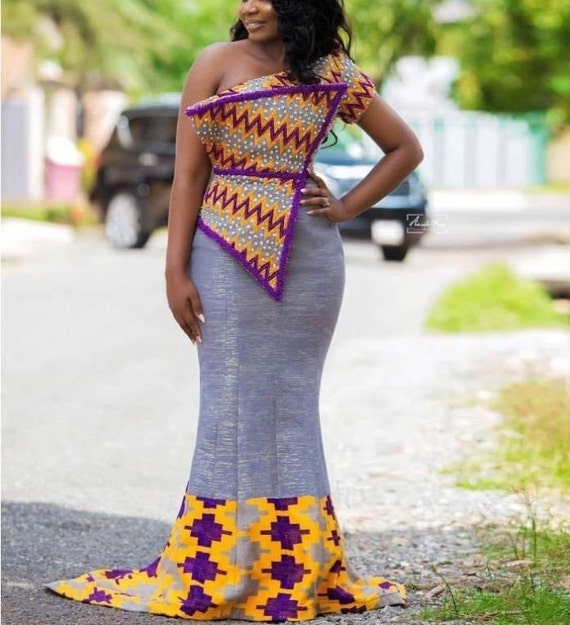This detailed color photograph showcases a confident black woman, who is striking a pose while modeling a contemporary, daring dress. The image is cropped to show her from the nose down, with her hand placed assertively on her hip, enhancing her feminine curves. The dress itself is a striking light lavender color, extending to the floor and covering her feet, giving it a sweeping and elegant effect. More vibrant hues of purple and yellow, interspersed with gray zigzag patterns, adorn the top of the dress and reappear towards the knees, adding bursts of color to the overall design. The dress has an intricate pop of purple and gold at the chest, further accentuating its bold style. The woman stands on a gravel road, with an out-of-focus black car and trees in the background, hinting at a suburban setting.